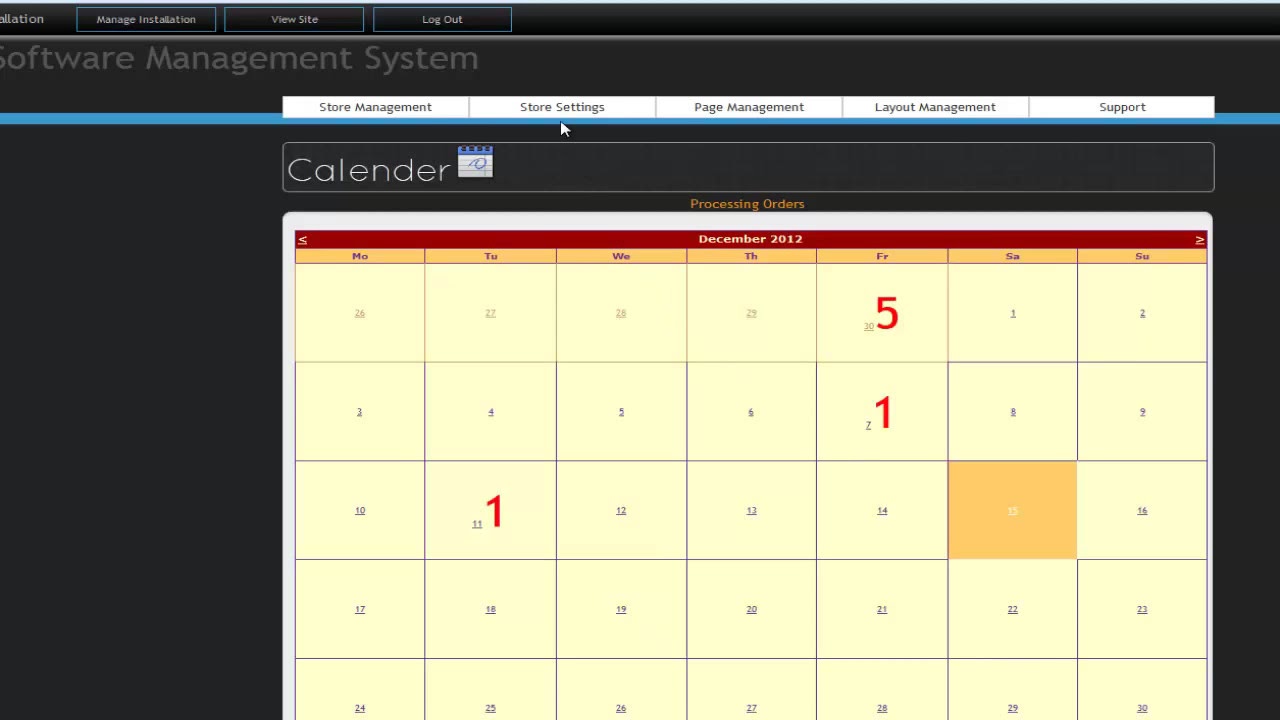The image depicts a screen capture of an online calendar from a software management system, serving a store management purpose. The calendar is primarily beige with a grid layout and is open to December 2012. The interface features a black background with several toolbars and buttons, including options for managing installation, viewing the site, and logging out. Below these are tabs labeled "Store Management," "Store Settings," "Page Management," "Layout Management," and "Support."

Prominently, there is a calendar section titled "Processing Orders," indicating possibly scheduled business activities. Key dates are marked with red numbers: a '5' on a Friday (Nov 30, 2012), and '1's on both Friday the 7th and Tuesday the 11th of December. Additionally, Saturday the 15th is highlighted in a darker orange color, suggesting it is selected or significant. The cursor within the screen capture implies that settings may be being adjusted, possibly from a video screenshot.